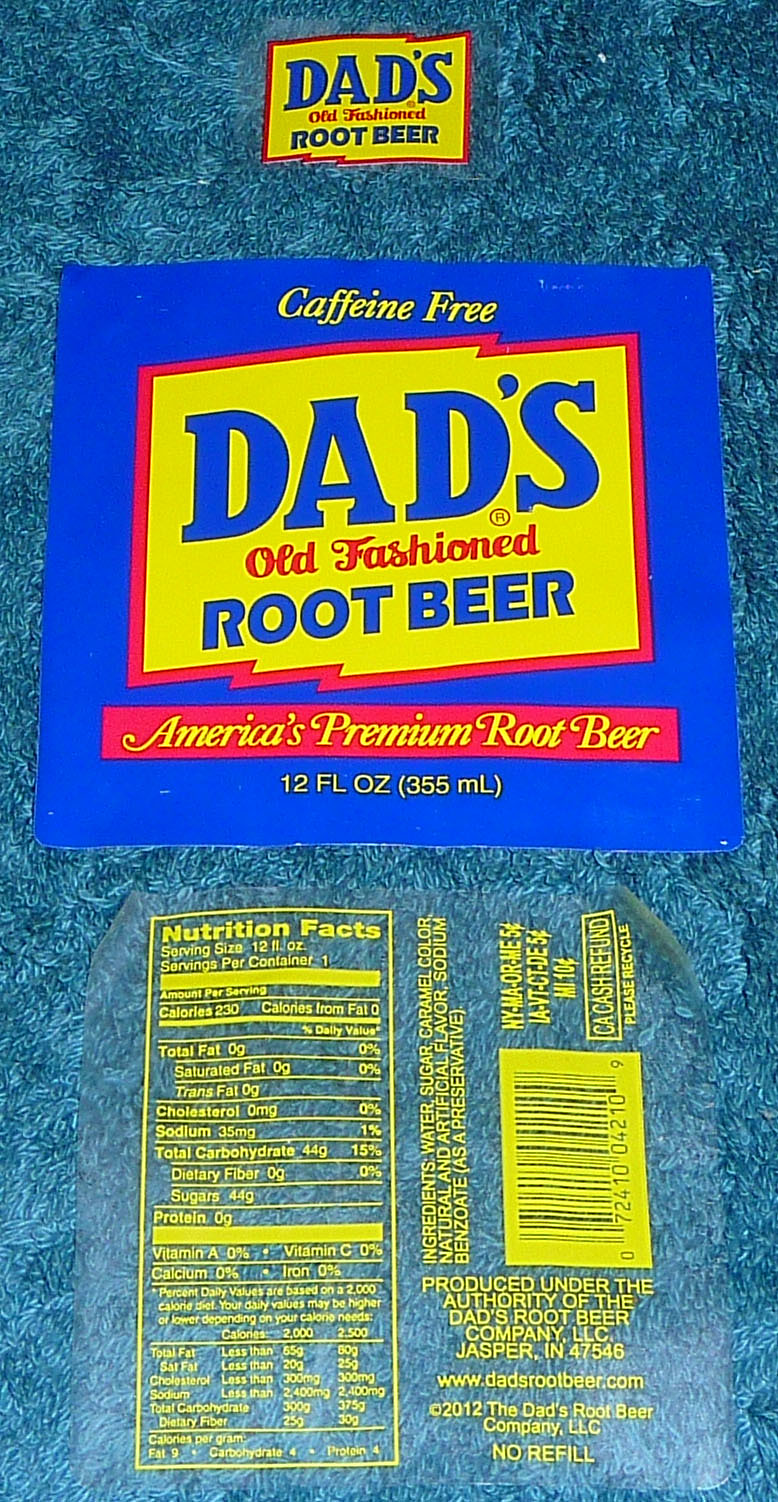In the photo, three distinct stickers are prominently displayed against a textured blue background that resembles either carpet or a towel. The top sticker is the smallest, shaped somewhat like a flag. It features a red outline surrounding a yellow background with blue and red text proclaiming "Dad's Old Fashioned Root Beer." 

The middle sticker is considerably larger, about twelve times the size of the top one, sharing a similar design. This blue square sticker carries the same flag-like motif with identical text: "Dad's" in blue, "Old Fashioned" in red, and "Root Beer" in blue, all set against a yellow background with a red border. Positioned above the flag design are the words "Caffeine Free," and below it reads "America's Premium Root Beer." 

The third sticker appears to be a nutritional facts label, typical of what you would find on the back of a root beer bottle, rounding out the trio of stickers featured in the photograph.